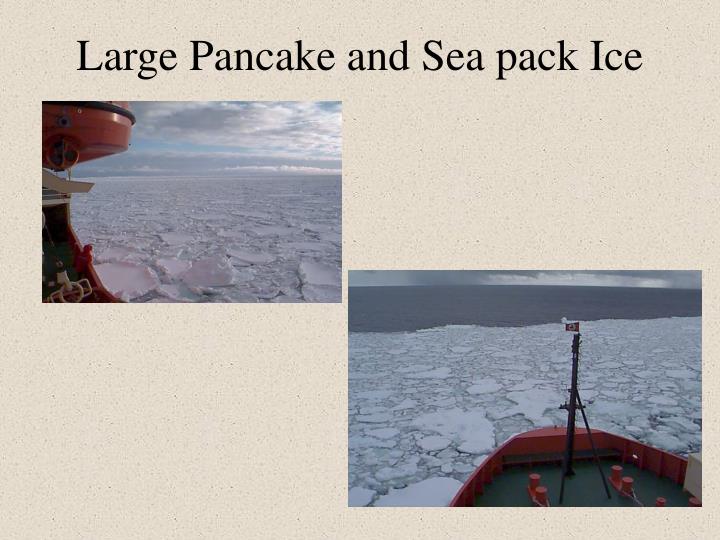This rectangular image, approximately six inches wide and four inches tall, features two distinct photographs set against a light brown, sandstone-like background with small dots. At the top, in bold black print, are the words "Large Pancake and Sea Pack Ice." 

The left photograph, located directly beneath the text, measures around two inches wide and one inch tall. It showcases the thick chunks of ice dominating the lower part of the image, while the upper portion reveals a blue sky dotted with thick white clouds. A part of a red ship or boat is visible on the left side of this photo.

The larger photograph, approximately three inches wide and two inches tall, is situated in the bottom right corner. This image captures the perspective from the front of a red ship with a green deck, as it attempts to navigate through the thick, broken ice. The ice extends up to the ship's bow, beyond which the water is dark gray and clear of ice. The outdoor setting during the daytime suggests a very cold environment where the water has partially frozen over.